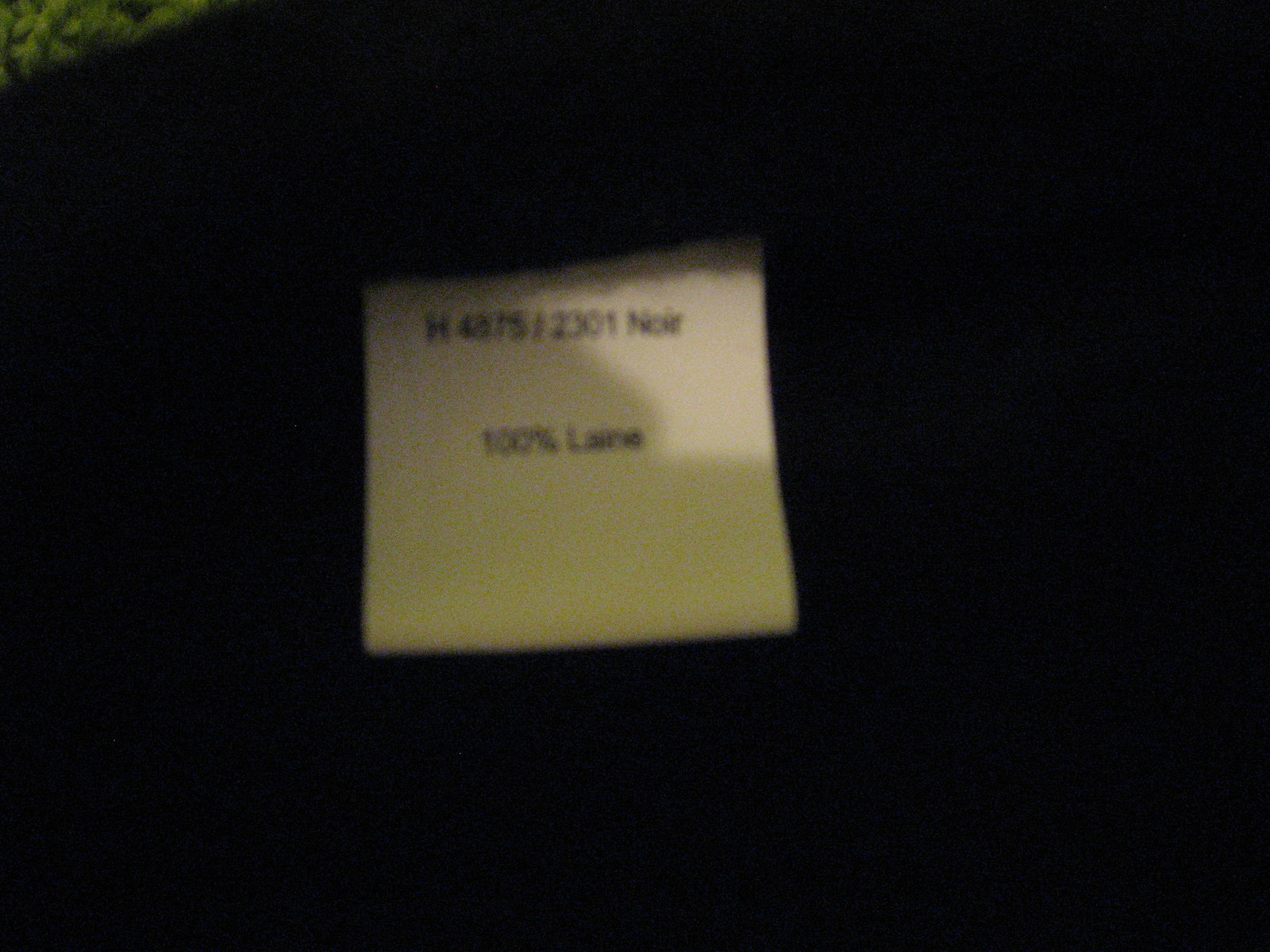This image features a slightly blurry clothing tag, set against a black background. The tag itself is a white square, with black text that is somewhat difficult to decipher. At the top, the text appears to read "NOR" or possibly "NOIR," written in a prominent black font. Below this, the text indicates "100%," followed by letters that seem to spell "L-A-N-E" or "L-A-R-N-E," though the precise wording remains unclear due to the blurriness. There is no additional text or markings visible on the tag. The tag's attachment to any garment is not evident in the image. In the top left corner of the image, a small patch of green can be seen adjacent to the black background, but no other details are present.